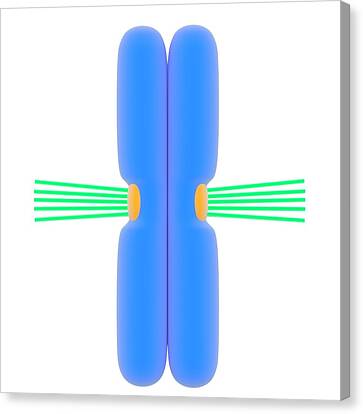The image depicts a piece of artwork centered on a white canvas with a gray, raised edge, casting a slight shadow against a white background, suggesting depth. Dominating the canvas are two tall, slender, vertical blue tubes touching side by side, appearing as mirror images of each other. In the middle of each tube, on the outward-facing sides, there is an orange or yellow oval (alternately described as a circle) from which green horizontal lines emanate towards the sides of the canvas. These green lines, reminiscent of sonar waves, give a dynamic quality to the artwork, enhancing its visual impact. The overall composition is minimalist yet vibrant, with the blue, green, and orange/yellow elements sharply standing out against the pure white background.